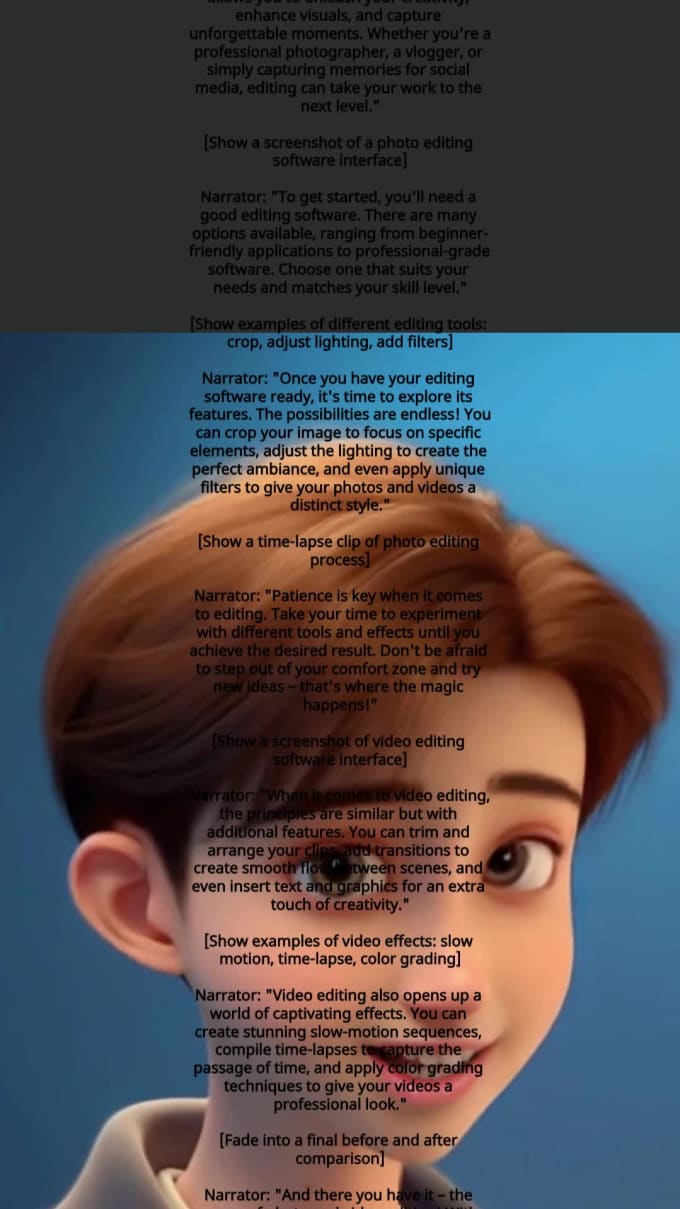This image features an AI-generated headshot of a young boy with short auburn hair and soft hazel eyes. He has delicate, Pixar-style features, including a gentle smile that reveals his teeth, and he's wearing a gray shirt. The background is teal blue and gray, divided into sections with small, printed black text that resembles a narrator's script for a software tutorial video. The text includes lines like, "To get started, you'll need a good editing software" and "Once you have your editing software ready, it's time to explore its features." The overall aesthetic combines animated facial characteristics with instructional elements embedded in the background.